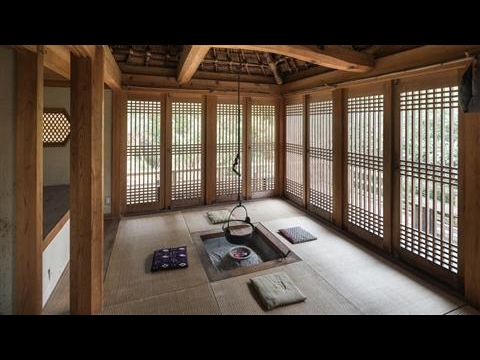The image depicts the interior of a traditional Japanese-style house, exuding a serene, Zen-like ambiance. Central to the scene is a suspended pot hanging by a string or chain from the wooden ceiling, directly over a square fire pit recessed into the wooden floor. Surrounding the fire pit are four cushions, one on each side, offering a cozy seating area. Various wooden elements dominate the architecture, including beams, panels, floors, and sliding doors, which let in natural light and offer glimpses of trees and daylight outside. The overall setup resembles what one might find in an old Japanese movie, combining functionality with rustic elegance. The room's traditional layout and materials emphasize a harmony with nature, characteristic of Japanese culture.